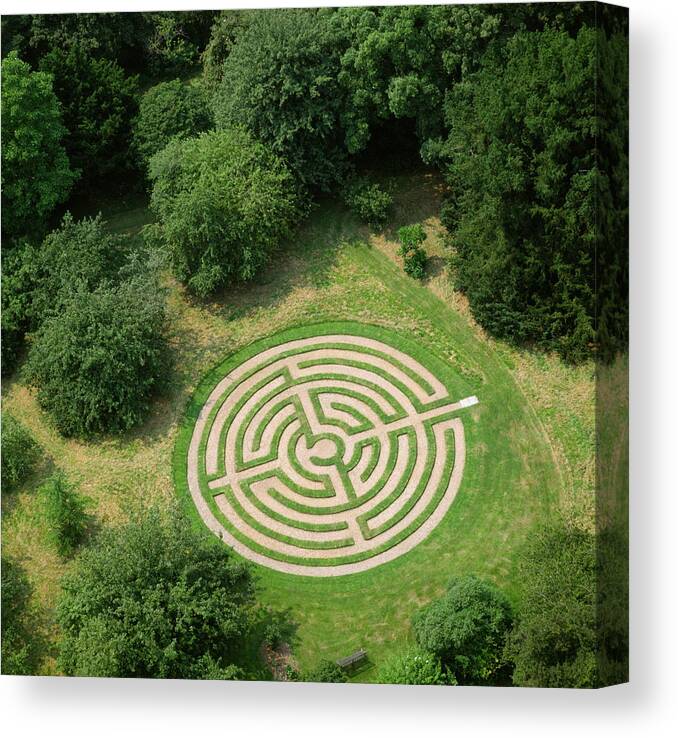This aerial photograph captures an open field featuring a meticulously designed circular maze at its center. The maze, which resembles a crop circle, is a striking combination of bright green grass pathways and brown walking trails, forming a complex pattern with various routes and dead ends leading towards the middle. The surrounding landscape comprises a lush, grassy area that transitions into dense, bushy woodland, creating a vibrant contrast between the cultivated and natural environments. Adding to the scene's intricacies, the bottom of the image reveals a faint outline of what could be a bench or a metal barbecue. Taken on a sunny day, possibly from a drone, this overhead image offers a unique perspective that emphasizes the maze's potential visibility from great heights, invoking a sense of otherworldly design.